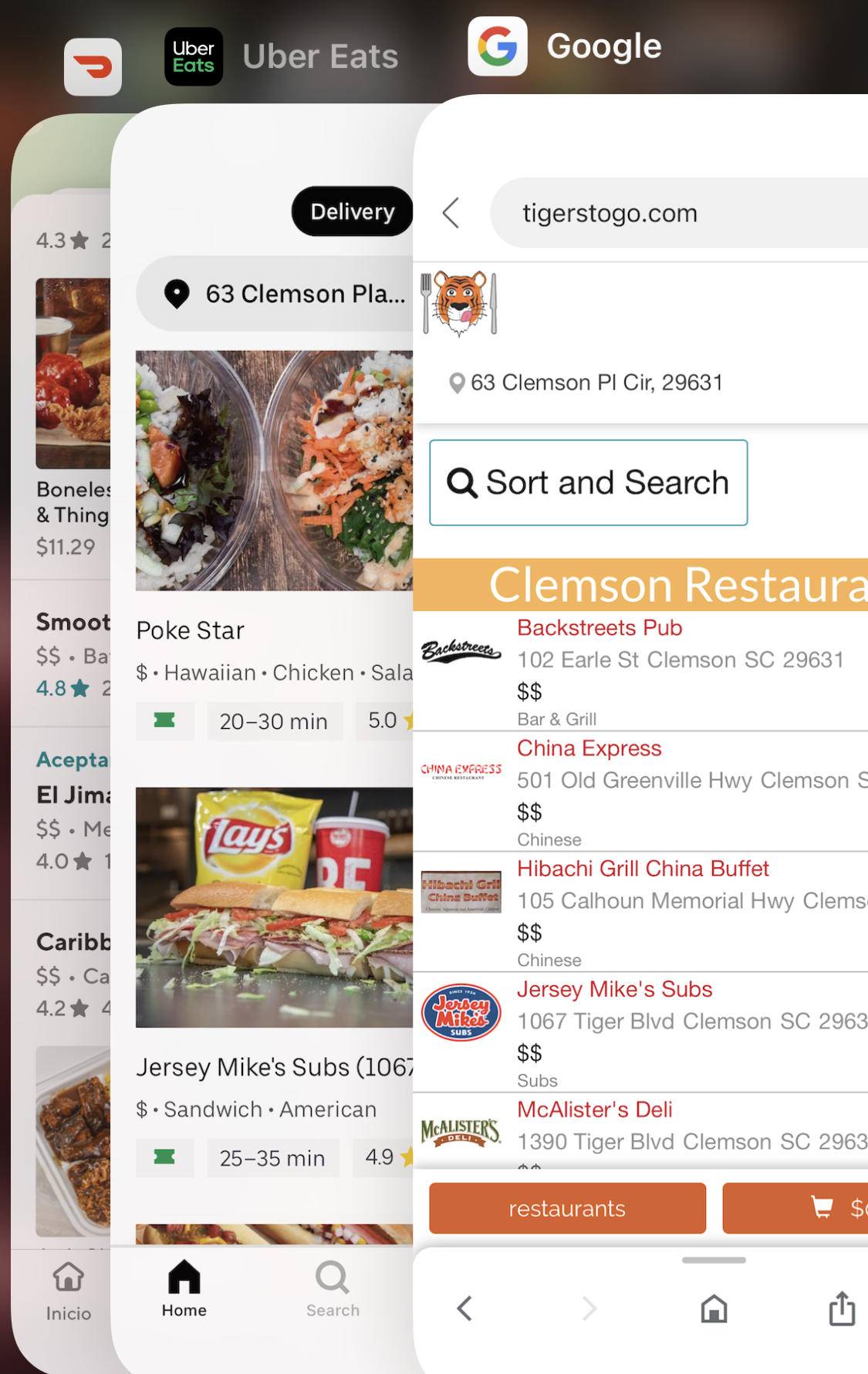This image showcases a multi-layered display from a cell phone screen, featuring three distinct applications: DoorDash, Uber Eats, and Google search.

In the topmost segment of the screen, the open Google search displays "tiger" and "tigers2go.com" in the search bar, along with the address "63 Clemson Place Cirque" and its corresponding zip code. There are options for sorting and searching. Below this search information are five distinct categories listing various restaurant options available in the Clemson area, likely for ordering food.

The middle layer reveals the Uber Eats app, focused on an interface facilitating food delivery. This section highlights locations pinned on a map, indicates delivery options, and includes pictures of food items such as Lay's potato chips and a beverage. There are also icons representing a search functionality and a black house symbol, possibly indicating the delivery address.

At the bottom layer, the DoorDash interface is partially visible. This section is less detailed but shows star ratings for restaurants and various images, likely depicting food items available for order.

Overall, the image encapsulates the navigation and comparison of food delivery options across different platforms on a mobile device.